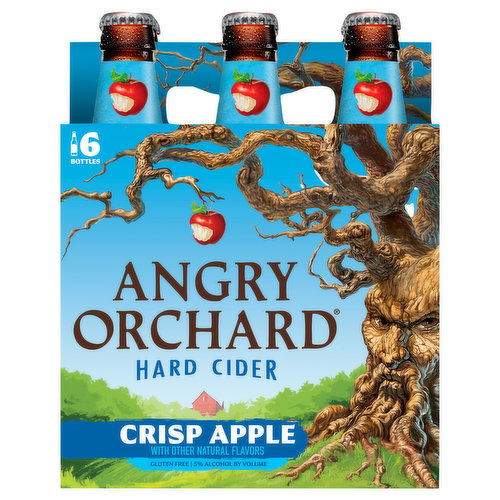The image depicts a vibrant product listing for a six-pack of Angry Orchard Hard Cider, specifically the Crisp Apple variety. The packaging sits against a transparent, thus white, background, emphasizing its product showcase nature. The front and visible side panels prominently feature the Angry Orchard logo, characterized by a vividly illustrated tree with a menacing face, slanted eyes, a lumpy nose, root-like beard, and branch-like hair. The tree holds a single apple with a bite taken out, hanging from a limb.

The upper left of the packaging declares "six bottles" in bold white text, while the brown and blue text below spells out "ANGRY ORCHARD" and "HARD CIDER" respectively. A blue band at the bottom reads "CRISP APPLE with other natural flavors" in white.

Three of the six bottles peek from the top, showing blue neck labels adorned with apples also bearing bites taken out. The carrying handle is visible behind them. The background of the packaging includes a bright turquoise sky, a red barn, and green foliage, adding to the product's vibrant and natural appeal. The label also mentions key product details such as being gluten-free and having 9% alcohol by volume.